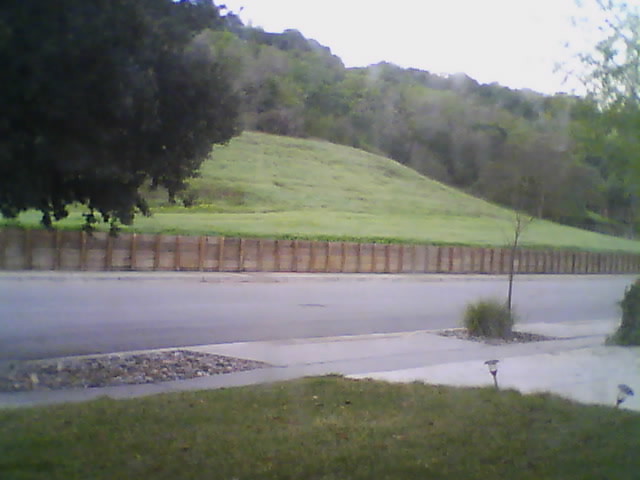In the foreground of the photograph, a lush expanse of grass is visible, exhibiting various shades of green—from darker to lighter tones, interspersed with hints of yellow-green areas. Dispersed across the grass, several black stick-like solar lights stand, each topped with a light fixture. To the right side of the image, a verdant green bush is surrounded by an assortment of rocks in hues of brown, gray, and off-white. On the opposite side, a similar rocky area is present. Beyond the grass and rocks, there's a light brown retaining wall. Behind this wall, a gently sloping hill is covered with multiple shades of green grass. Dominating the scene is a large, dense, dark forest-green tree, standing in front of a substantial tree line that stretches across the background. Above the tree line, a portion of the sky is visible.